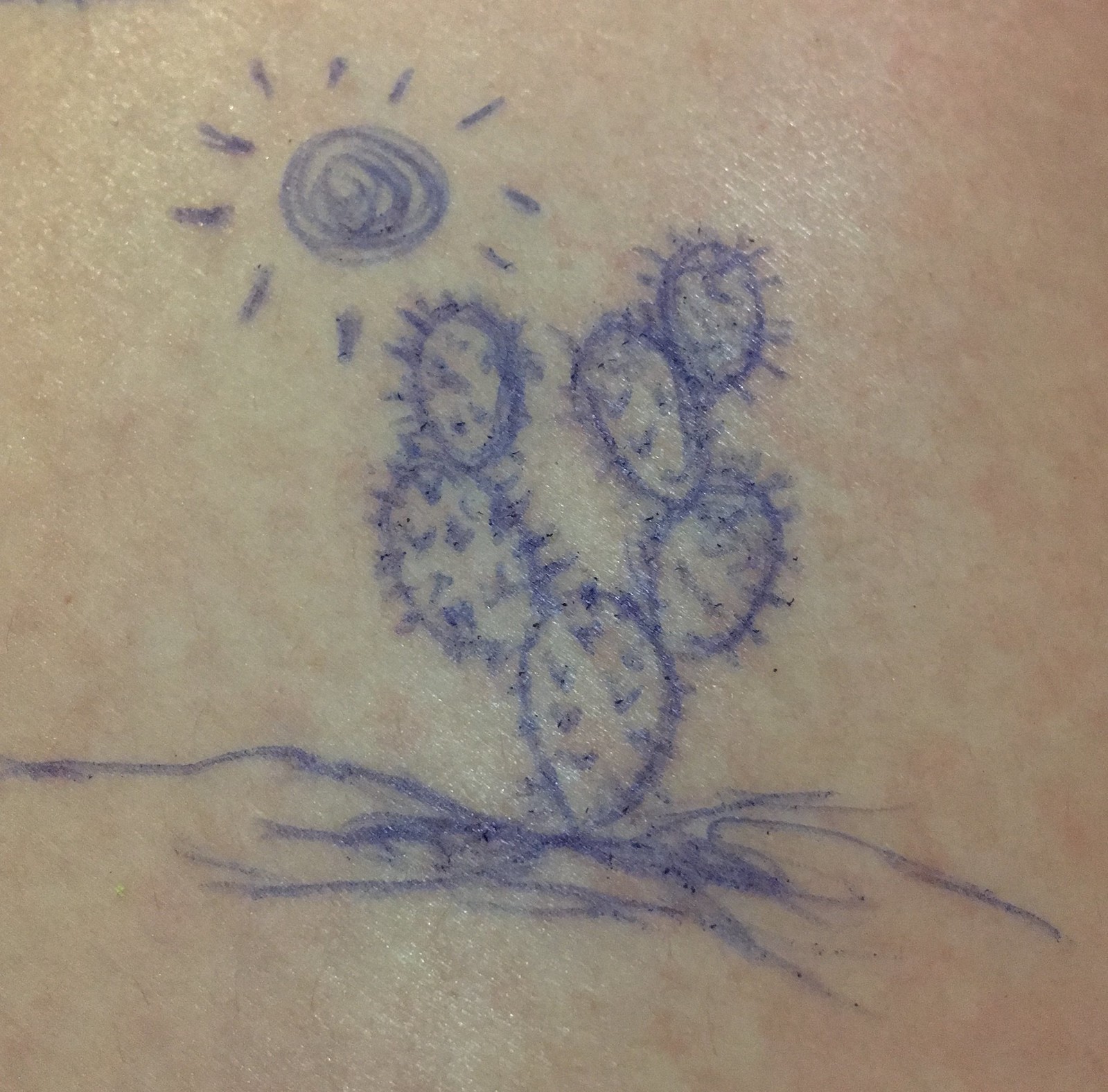This is a highly detailed close-up color photograph of a light-skinned person's body, showcasing a hand-drawn sketch that resembles a simplistic tattoo created with a blue ballpoint pen. The photo captures the delicate texture and natural tones of the skin, emphasizing an intimate and personal perspective.

Prominently featured just off-center towards the top left is a scribbled blue circle representing the sun, with irregular lines radiating outward in all directions. Below the sun and towards the bottom right is a stylized depiction of a cactus made up of ovals interconnected to form the classic, branching cactus shape. The central oval has small 'v' shapes around it to mimic cactus spines, and it branches out with additional ovals stacked in various directions to the left and right, creating a visual impression of a desert plant. Beneath the cactus, horizontal lines and scribbles evoke the appearance of a dry, desert-like landscape, adding depth to the sketch.

The image strikingly combines artistic elements with the raw, natural look of human skin, making it appear almost like an ephemeral piece of body art rather than a permanent tattoo.